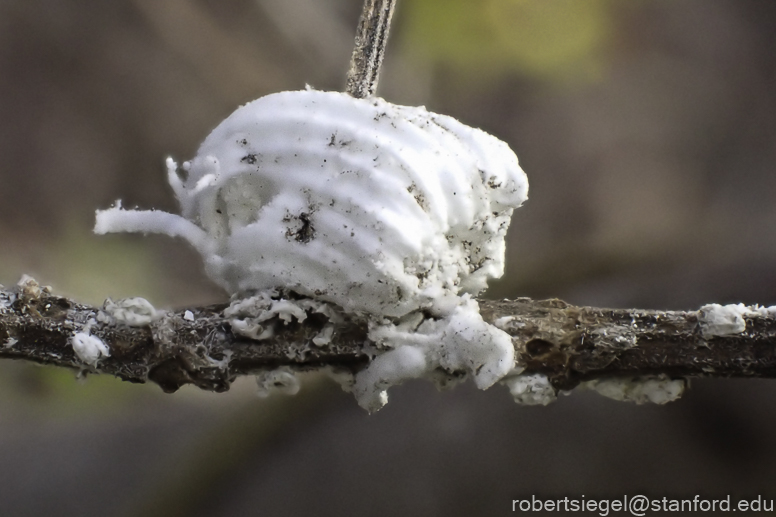The image is a detailed color photograph in landscape orientation, featuring a prominent brown stick that runs horizontally across the frame. This stick is dotted with small white patches of what appears to be fungal growth. The most significant feature is a large, puff-like scoop of white material, which is bulbous and resembles a melted marshmallow or foamy fungus, resting prominently in the center. This central mass has subtle fluted lines and a structure akin to an antenna protruding from its left side. There are also minor protrusions that might be legs or attachments to the stick. Another intersecting branch runs upwards through the top center of the image, blending seamlessly into the out-of-focus background, which is a soft, mottled mix of dark purple and gold tones. A yellow blob is faintly visible near the top of the image. The photograph carries an air of photographic realism, with extensive focus on the main subject. A discreet white watermark reading "Robert Siegel, robertsc at stanford dot edu" is located in the bottom right corner.